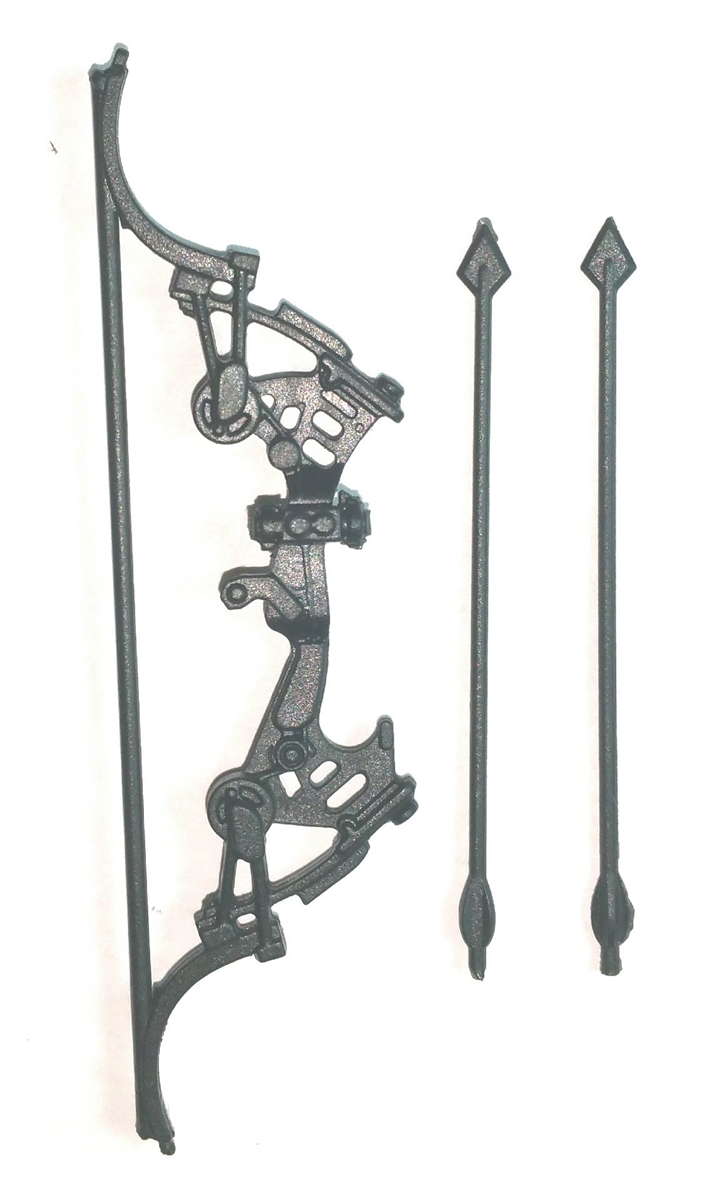The image depicts a highly detailed, stylized compound bow and two arrows positioned to the right of it. The arrows feature diamond-shaped arrowheads and appear to be crafted from a single material, possibly plastic, resin, or cast iron, with metal-like feathers. The compound bow, predominantly gray and resembling cast iron, includes intricate design elements such as cams, pulleys, and cylindrical components. The bow's main structure showcases several cut-out slots, levers, and a slight curve at the bottom. Notably, it lacks a traditional bowstring, instead having an iron bar where the string would typically be. The craftsmanship, characterized by multiple gears and articulations, lends a steampunk aesthetic to the piece, indicating a modern interpretation rather than an ancient artifact. The overall impression is that of a finely detailed model, potentially miniature, yet exhibiting sophisticated engineering elements typically challenging to replicate on a small scale.